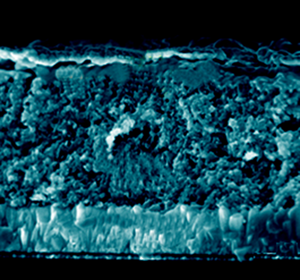This image features a highly detailed, close-up section of an object against a black background, with black areas framing the top and bottom. The primary material showcased appears rocky and varies in color and texture, primarily presented in multiple shades of blue. 

At the bottom, the material has a light blue hue, resembling ice, and extends upwards where it transitions into darker blues. These dark blue areas exhibit a more rocky appearance interspersed with lighter blue regions and white spots, some of which are central and towards the bottom right. Moving further up, the texture continues with a mix of lighter and darker blues, giving the impression of varying depth and ruggedness.

Toward the top of the image, the colors become swirly with thin, light blue lines interspersed with white areas that appear almost cloudy. The object’s texture throughout suggests it might be a cross-section of a diverse, visually complex material, potentially resembling natural or microscopic structures, with undulating, bumpy, and grooved features. Despite its abstract qualities, the object is mostly dominated by turquoise, dark blues, and white, adding to its intricate and layered appearance on the black background.